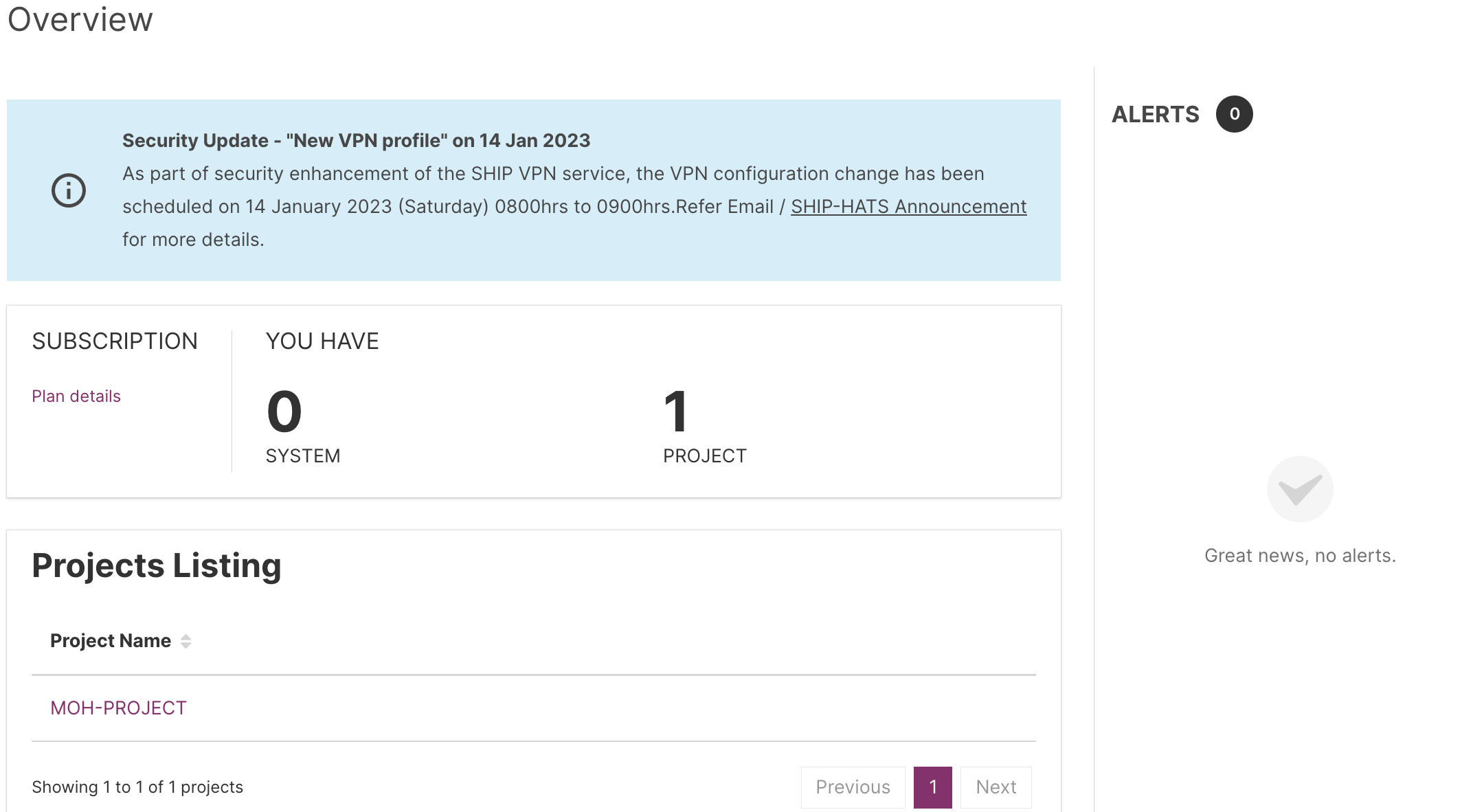On a white background, the top left corner features the word "Overview" in black text. Below it, there is a light blue square with a black circle containing the letter "I" on its right side. To the immediate right, the text reads "Security Update: New VPN Profile on 14 January 23." In lighter black text below, it states, "As part of the security enhancement of the ship VPN service, the VPN configuration change has been scheduled on 14 January 23, Saturday, from 0800 hours to 0900 hours, for email."

Further down, an underlined text says "ship-hats-announcements," followed by non-underlined text that reads "for more details." On the right-hand side, there's a white button with black text labeled "Abort" next to a black circle containing a white zero. Beneath the light blue square, the word "Subscription" appears in black text, with "Plan Details" in blue underneath.

Toward the right, it indicates you have "zero systems" and "one project." At the bottom, under "Project Listings," it lists the project name "MLH-project," followed by text stating "showing 1 to 1 of 1 projects." On the right-hand side, the word "Previous" appears in gray, followed by a purple box with a white number one, and the word "Next" also in gray.

Centrally to the right, a gray checkmark is present with the text "Great news, no alerts," written underneath in gray.